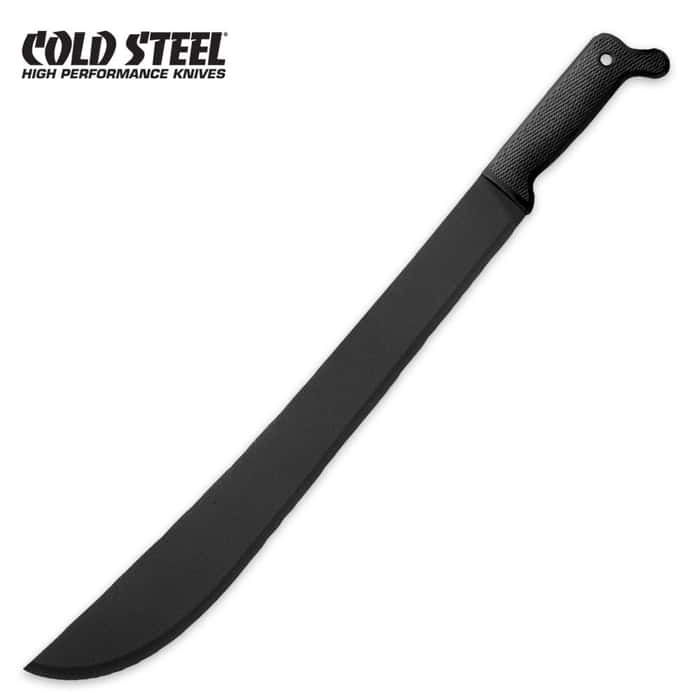The image is a square black-and-white photograph of a large, black machete. The machete's handle begins in the upper right corner of the image, identifiable by a hole and a small angled nub at its end, and continues diagonally until the blade terminates at the bottom left corner of the frame. The handle, likely made of plastic, features a diagonal design and a screw securing it to the blade. The entire machete, including the blade's edge, is uniformly black. The background has been removed, leaving the machete to prominently float against a white backdrop. In the upper left corner, the text "COLD STEEL" is printed in a hand-drawn, all-caps font, followed by "HIGH PERFORMANCE KNIVES" in smaller capitalized letters below. The photograph combines elements of representationalism and realism, enhanced by the stark contrast between the black machete and the white background.